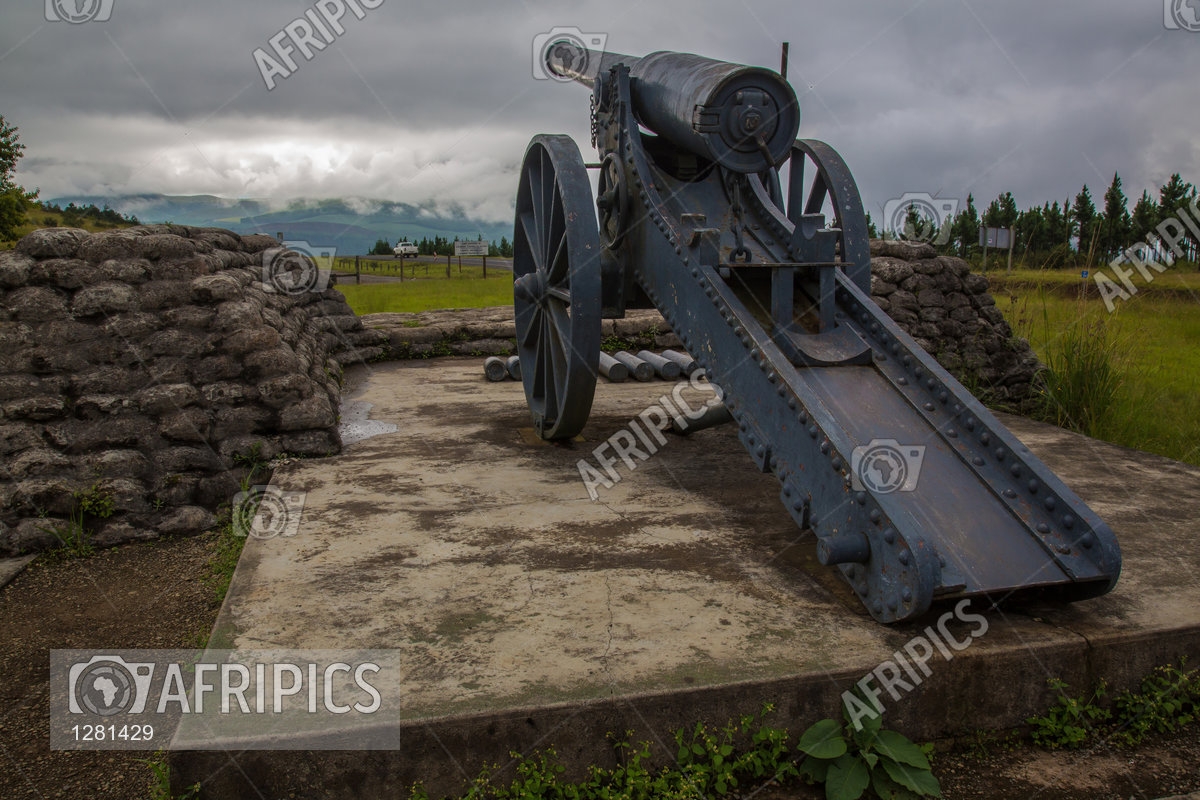The photograph captures a large, historical cannon mounted on wheels, situated on a rectangular stone or concrete pad with several projectiles lying in front of it. The cannon, made of heavy steel painted blue-gray, features riveted metal and an 8-inch barrel. Surrounding the cannon, sandbags are stacked higher on the left and right sides than in the front, forming a protective barricade. The scene is set in an open, green field with green valleys and hills visible on the distant horizon. The sky overhead is dark and cloudy, suggesting an impending storm. Cedar trees border the sides of the field, adding to the depth of the landscape. The photograph bears multiple AfriPix watermarks across it, along with the text "AfriPix 1281429" prominently displayed. In the background, a fence line suggests that this might be private property, possibly a farm.